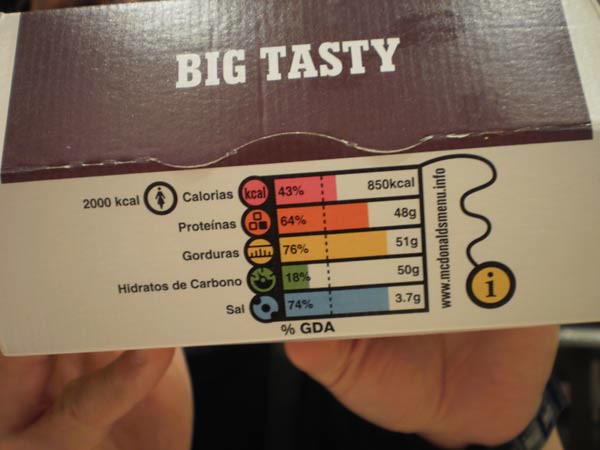A close-up photo features a pair of hands, likely male owing to their larger build, though gender is indeterminate, holding up a rectangular box. The skin tone of the hands is light. The box has a brown lid adorned with white lettering that reads "Big Tasty." The side of the box, which is prominently faced towards the camera, displays nutritional information. It notes that the contents provide 850 calories, which constitutes 43% of a 2,000 calorie daily diet. Additionally, the box offers details on protein and other nutritional values, structured in a color-coded format. The information is written in Spanish, adding to the box's detailed presentation.